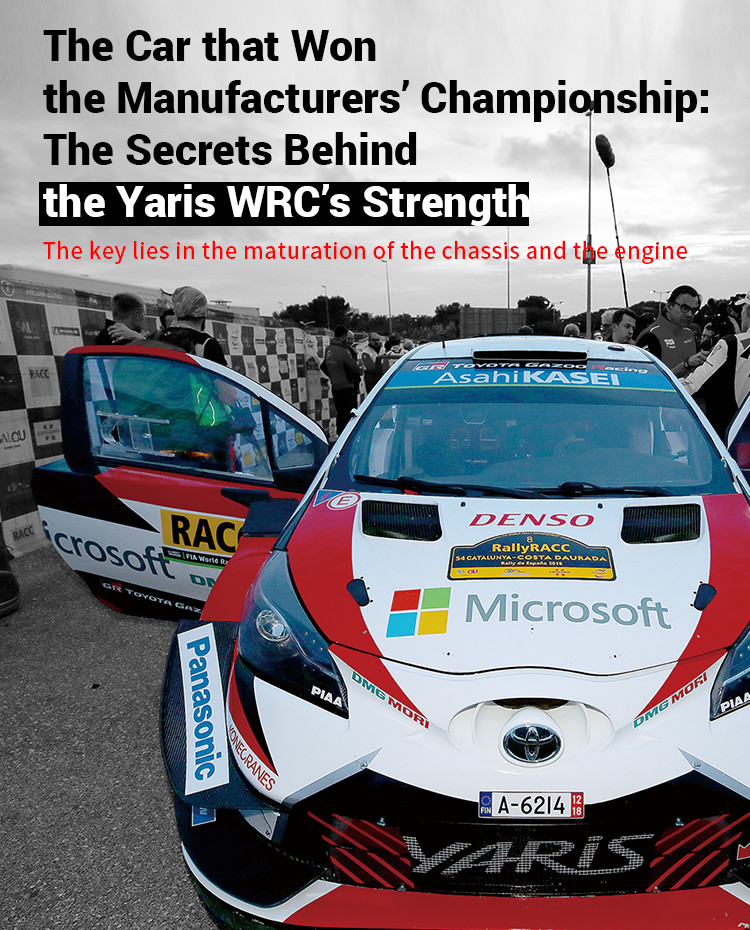The photograph is a vertically rectangular, full-color image with added text, captured outdoors under natural light. The image features a red and white race car, identified as a Yaris, prominently positioned in the center with both doors open, but no one inside. The hood of the car displays several sponsor logos, including Denso, Bally, RACC, and Microsoft. The license plate on the front reads "A-6214" with "Yaris" below it. Surrounding the car, the background, including the sky, trees, and people, is in black and white, contrasting starkly with the vibrant colors of the car. The top of the image features a headline in black text that reads, "The car that won the Manufacturer's Championship: The secrets behind the Yaris WRC's strength." Below the headline, in white text with a black highlight, it states, "The key lies in the maturation of the chassis and the engine." To the left of the car, additional advertisements such as Panasonic can be seen, while racers and interviewers are visible to the right.